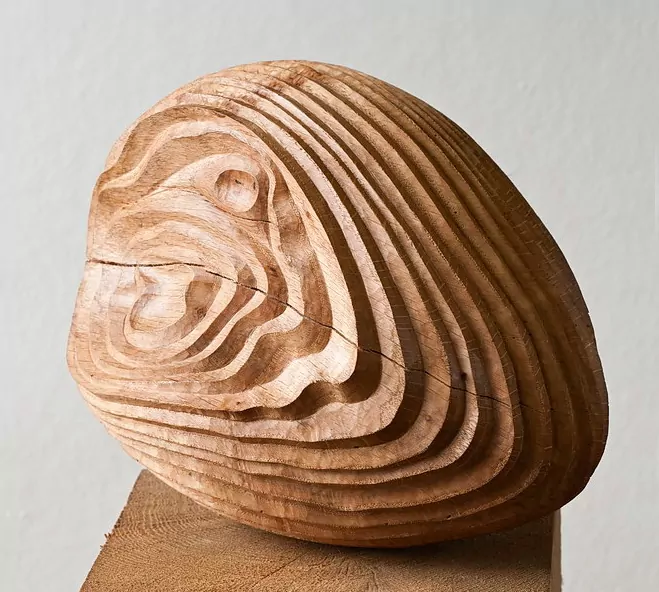This photograph depicts an intricately carved wooden sculpture resting on a smooth, square-cut wooden pedestal. The background is a gradient of light gray from top to bottom. The sculpture itself is walnut-shaped, wider at one end, and features rows of grooves and ridges that wrap around it in a circular pattern. The front displays a more detailed and elaborate carving, with additional indentations. A prominent horizontal crack runs through the middle, suggesting age or damage. The lighting highlights the left side of the sculpture, casting a subtle shadow to the right.